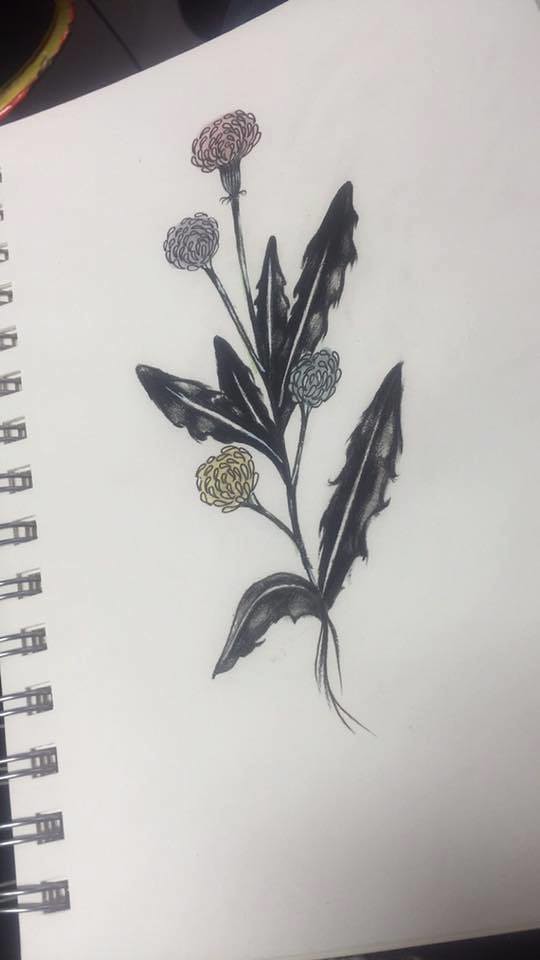This is a detailed illustration of four delicate flowers, drawn on the pages of a ring-bound notebook with blank white sheets. The silver rings of the binder, approximately a dozen in number, cut through square openings along the left edge of the page. The notebook rests on a wooden countertop, and at the top left corner of the image, a hint of a reddish-yellow bowl is visible.

The four flowers depicted in the illustration appear to belong to the same species but vary in color—one pink, one purple, one blue, and one yellow. These flowers feature very delicate petals and are clustered together, emerging from the same base. Their long and slender green stems converge into a set of loose, flowy roots. The plant also has six leaves, dark green to nearly black in color, resembling feathers in their shape. The artistic details capture the fragile beauty of the flowers and the organic texture of their foliage.